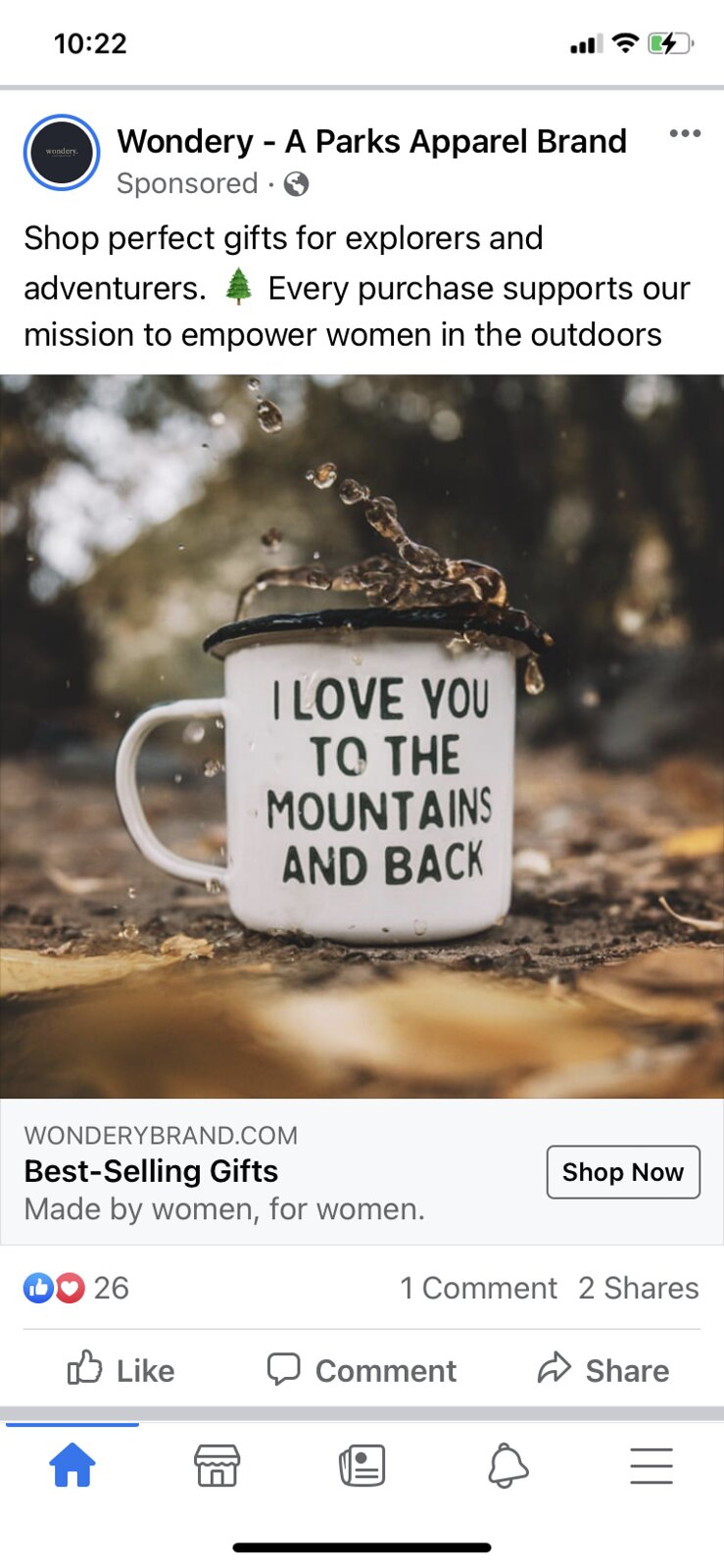**Instagram Ad for Wondery, a Parks Apparel Brand**

This advertisement, screenshotted from a phone at 10:22, showcases a beautiful image from Wondery, a parks apparel brand, tailored for social media enthusiasts. In the top left corner, the time is displayed, with battery, signal, and Wi-Fi status icons on the right. Below, a sleek interface features a black circle with a blue outline, followed by "Wondery - A Parks Apparel Brand" and a "Sponsored" label beneath.

The main post urges viewers to "Shop Perfect Gifts for Explorers and Adventurers," emphasizing that "Every purchase supports our mission to empower women in the outdoors." The attention-grabbing photo centers on a white coffee mug, adorned with the touching phrase, "I love you to the mountains and back." This mug rests on the ground amidst scattered leaves, with a creatively blurred background hinting at mountains and trees, enhancing the focus on the product.

Below the image, text highlights "Best-Selling Gifts" with the URL "WonderyBrand.com" and a "Shop Now" button to the right. Social interaction metrics show 26 reactions, one comment, and two shares, with standard engagement options like Like, Comment, and Share buttons available. The footer icons for Home, Marketplace, News, Notifications, and Menu ensure easy navigation.

Wondery celebrates women by offering thoughtfully designed gifts that encourage exploration and adventure in the great outdoors.